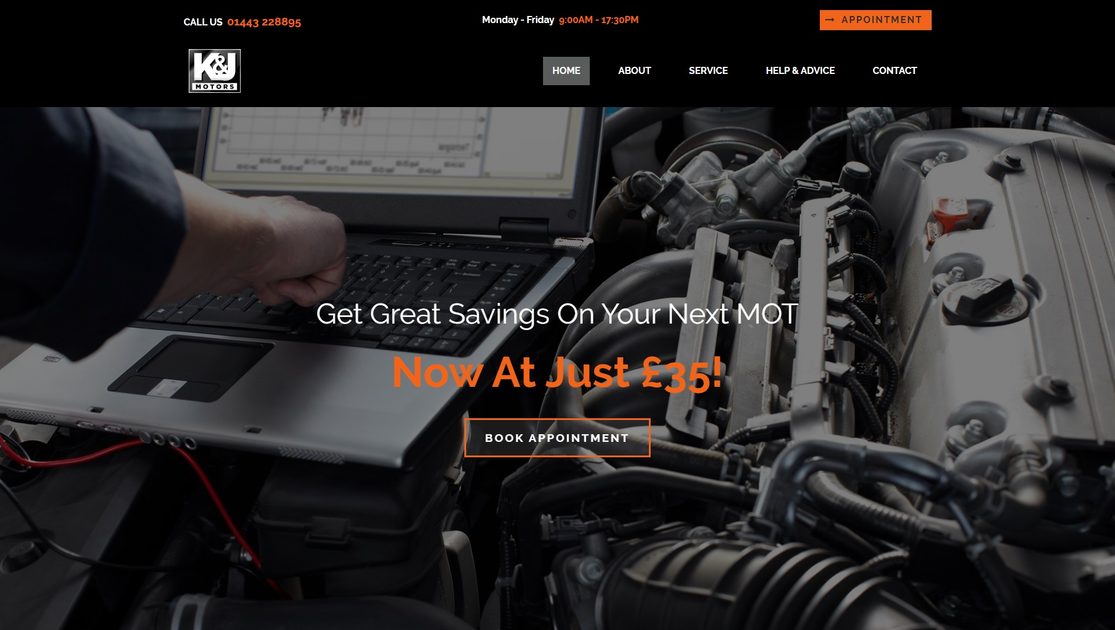This is a landing page for a motor center featuring a prominent logo that reads "K & J" at the top. The menu strip at the top is black with white text, displaying the following options: Home, About, Service, Help and Advice, and Contact. There is an orange button above the menu labeled "Appointment."

The main section of the page showcases a large picture of an engine, accompanied by a laptop computer with a man's hand interacting with it. Overlaying this image is a bold white text slogan that reads, "Get Great Savings on Your Next MOT, Now Just £35." Below this text, there is a button labeled "Book Appointment," inviting users to take action.